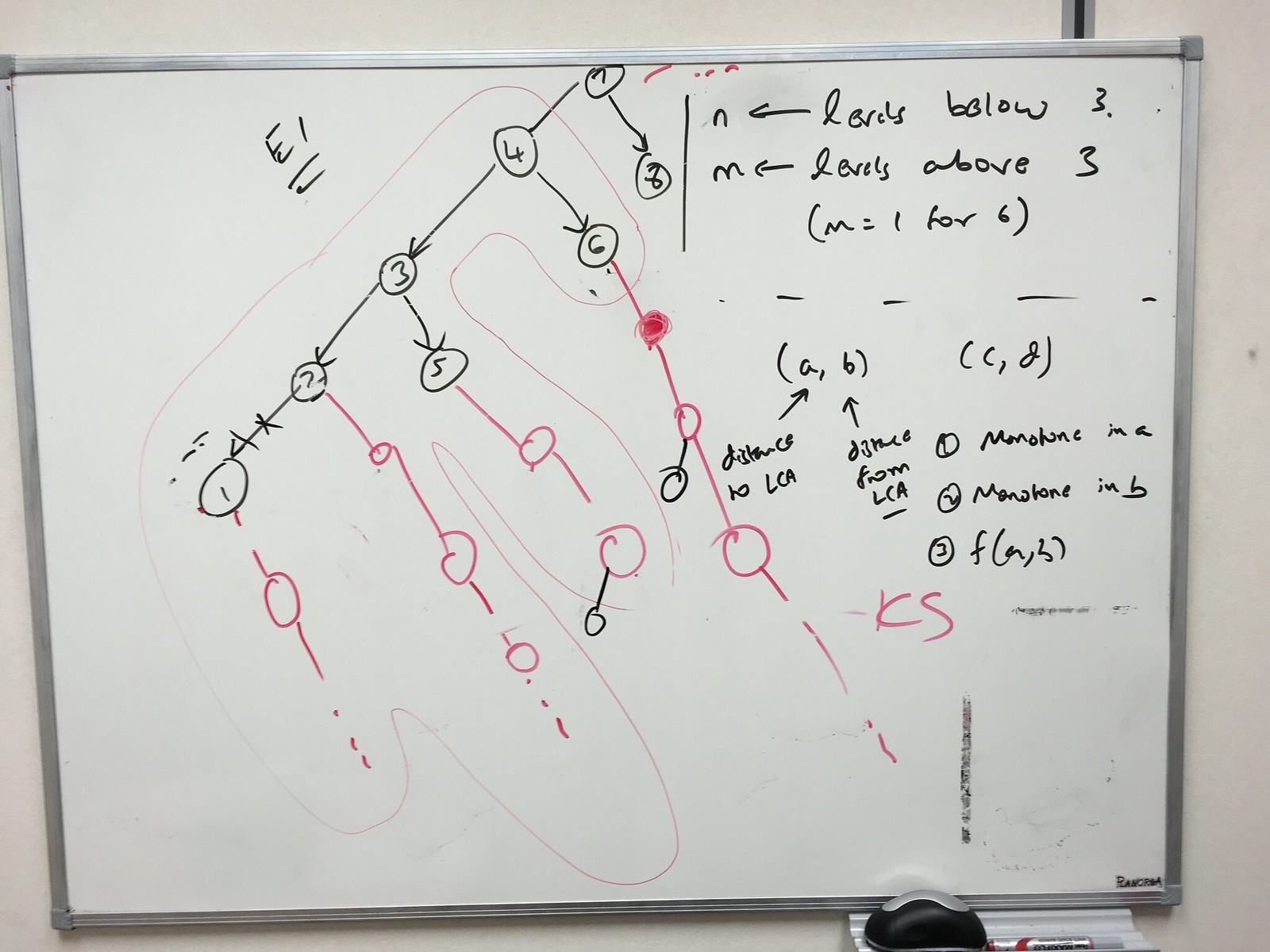This image features a whiteboard mounted on a white wall, encased in a sleek silver frame. At the bottom right corner of the whiteboard, there is a small tray containing a red and silver marker, as well as a black and silver eraser. The whiteboard is covered with detailed writing in both black and red ink.

On the top left corner, "E1" is written in black ink and underlined twice. Several numbers (1 through 8) are circled, each with an arrow pointing to the subsequent number. Directly below these numbers are red dashes with corresponding red circles, indicating different quantities: 

- Number one has one circle.
- Number two has three circles.
- Number five has two circles.
- Number six has three circles.

On the right-hand side of the board, additional information is written in black ink, including "N" followed by an arrow and the phrase "levels below three." Additionally, it states "M" with another arrow and "levels above three", and further clarifies with "M equals one for six." Below this, there are four black dashes, followed by text in parentheses reading "(A, B)" and "(C, D)." Further writing is present below these symbols, though it is less clearly defined in the description.